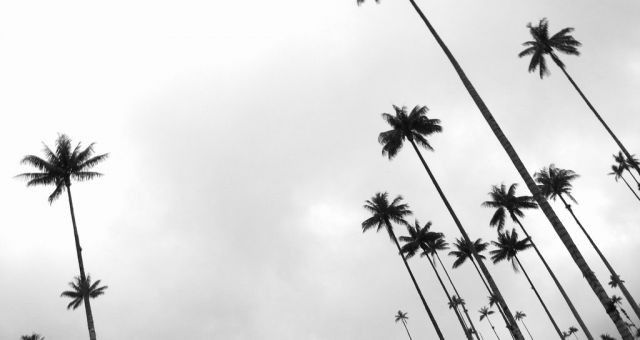This black and white photograph captures a foggy, cloudy daytime scene, looking upwards towards the sky. The image showcases a series of tall, healthy palm trees. On the far right, there's a dense cluster of palm trees, with one significantly taller than the others, their trunks climbing upwards and leaves fanning out at the top. On the left side of the frame, two additional palm trees stand tall, their tops also reaching toward the cloudy gray sky. The overall composition emphasizes the height and abundance of the palm trees against the overcast backdrop.